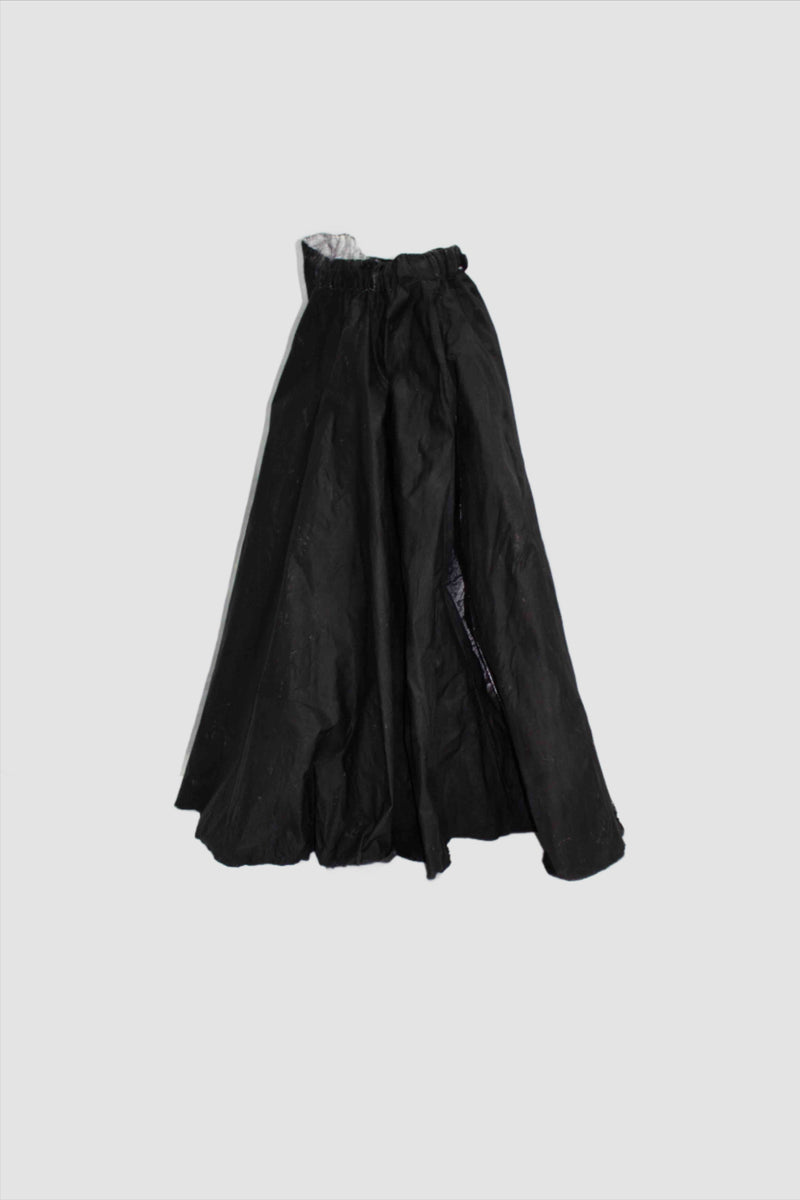The photograph depicts a black, floor-length skirt or the lower half of a dress set against a stark white background. The setting consists of a white floor and a white curtain backdrop with subtle wrinkles, contributing to an elegantly simple and minimalistic aesthetic. The black skirt appears to stand on its own, seemingly unsupported with no visible mannequin or stand, although there is a faint indication of an elastic band and possibly a subtle support from below. The skirt, wrinkled and possibly pleated, extends from the waist to the ankles of an average person, creating a striking contrast against the white surroundings. This carefully composed image exudes a sense of high fashion, suggesting its suitability for magazine features or other sophisticated displays.